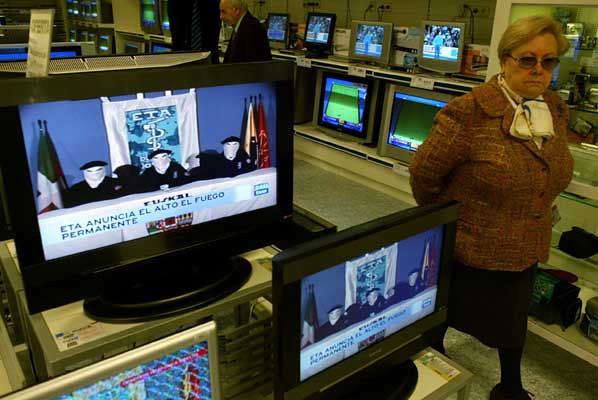The photograph captures an indoor scene at an electronics store, specializing in television sets and computer monitors, some of which appear to display content in Spanish with a headline reading "ETA enuncia el alto, el fuego permanente" against a blue background. The focal point is a middle-aged woman with short blonde hair, wearing sunglasses, a tweed jacket in an orangish-brown hue, a cream-colored blouse with a bow tie, a black skirt, and black stockings. She is walking through the dimly lit store, browsing the array of electronics displayed on pale yellow or beige shelves. In the background, an older man dressed in a dark suit with a white collar and balding grey hair wanders through the aisles, adding to the sense of a busy retail space. The overall ambience suggests a slightly dated atmosphere, with an assortment of reasonably flat screen televisions and monitors showcasing various channels, enhancing the impression of an electronics shop from a recent past era.